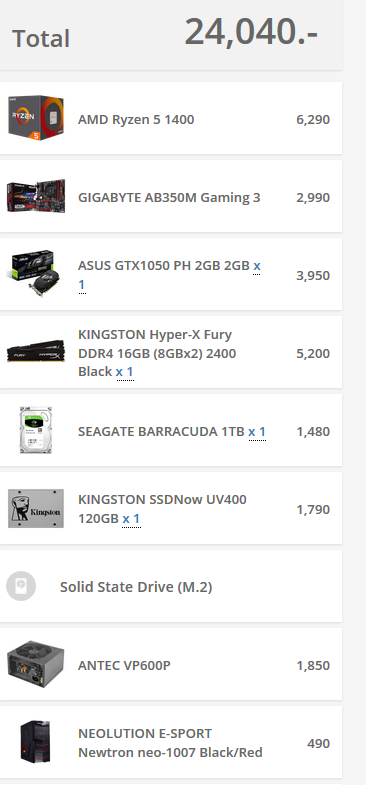A detailed screenshot from a cellphone showcases an organized list, likely related to gaming hardware. The background is a uniform gray, contrasted by white rectangles containing various items. At the top of the screen, the word "Total" is displayed on the left, followed by a value of "24,040" on the right, next to the word "Period" and a dash. 

Each rectangle below is structured with a picture of an item on the left, the item's name in the center, and a numerical value on the right. These values predominantly fall within the thousands range, suggesting they might represent points, but there are no dollar signs, indicating it's not monetary. The lowest value displayed is 490, located in the bottom right-hand corner.

The items listed from top to bottom include:
1. AMD Ryzen 5 1400
2. Gigabyte AB350M Gaming 3
3. ASUS with a series of numbers and an 'X'
4. Additional items follow, making up a total of nine entries.

Notably, one entry, "Solid State Drive M2," deviates by lacking numerical data. This meticulous arrangement allows for easy comparison and reference, underscoring the high level of organization on the screen.